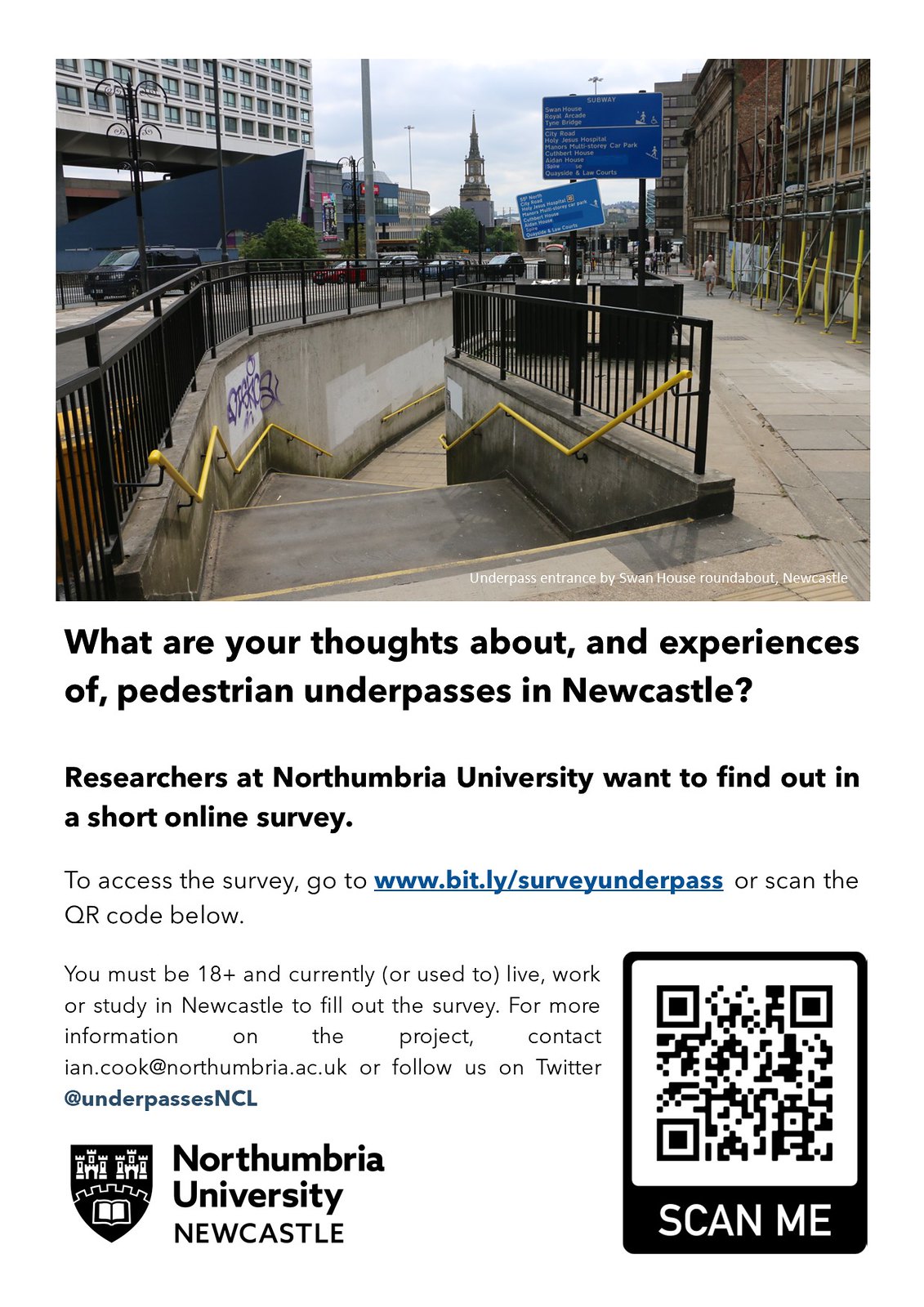The vertical rectangular poster features a photograph at the top and extensive text below. The photo showcases a staircase descending next to a road in an urban area of Newcastle, with a sidewalk on the right and buildings lining the street. Directly below the photo in bold black letters, it reads, "What are your thoughts and experiences of pedestrian underpasses in Newcastle?" Smaller text underneath states, "Researchers at Northumbria University want to find out in a short online survey." Additional details provide a link to the survey and a QR code for easy access. The bottom text also specifies that participants must be 18+ and currently, or have previously, lived, worked, or studied in Newcastle to participate. In the lower left corner is the Northumbria University Newcastle logo with a shield. Contact information and social media details are provided for further inquiries.